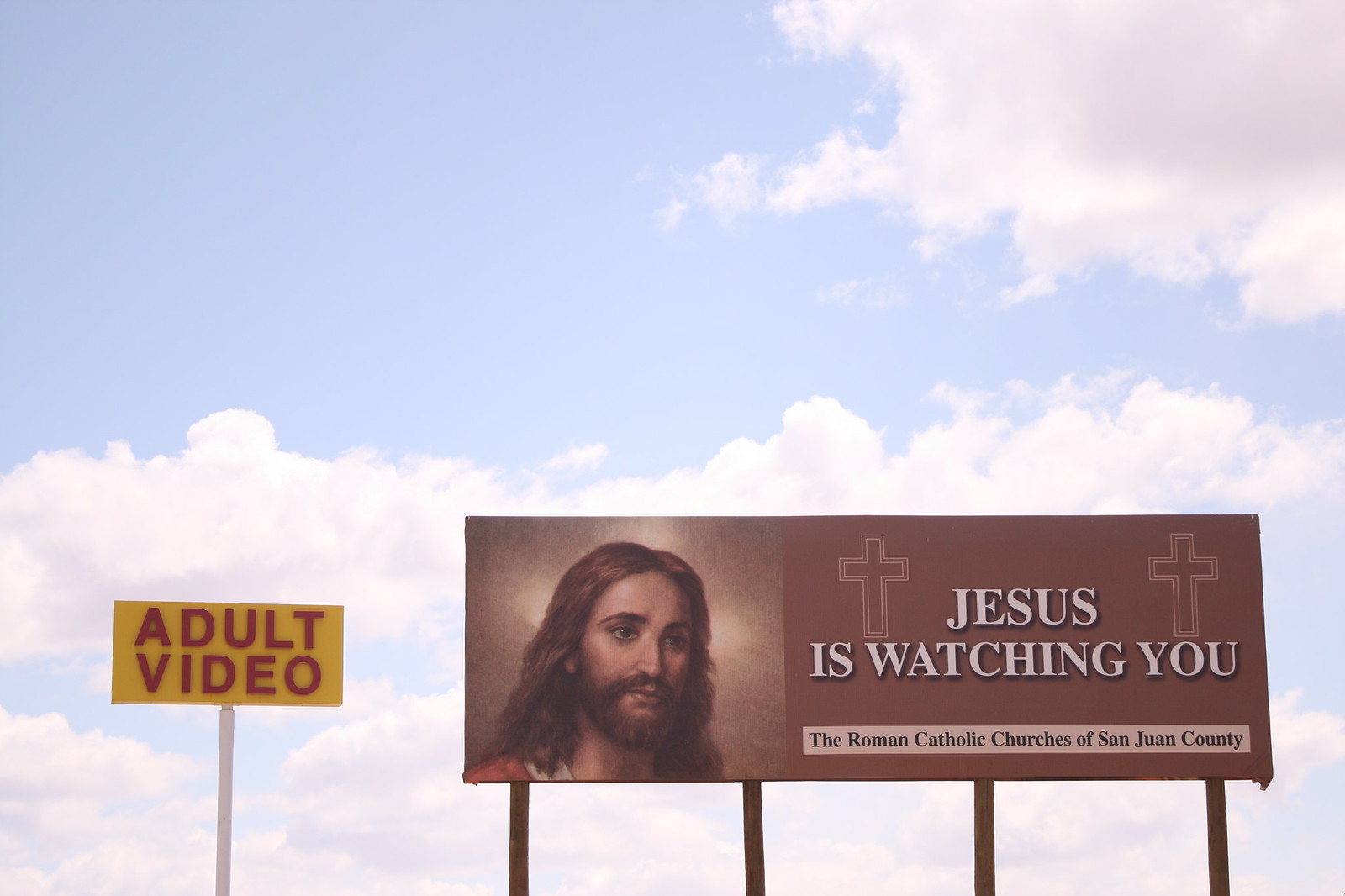In this rectangular landscape image, approximately 50% wider than it is high, two prominent signs command the viewer’s attention against a backdrop of a light blue sky dotted with white clouds concentrated towards the upper right corner.

On the left side of the image, a sign stands tall, starting roughly 20% into the frame. The sign, held by an unseen white pole, features a yellow rectangular background with bold red capital letters that read "ADULT VIDEO," reminiscent of McDonald's color scheme. The sign proportions are slightly more than twice as wide as it is high.

To the right of this sign, almost spanning from just left of the middle of the image to the far right edge, is a much larger billboard supported by four brown posts that are also not visible at their base. This billboard, framed in a brown background, presents an impactful and contrasting message with the text "Jesus is watching you." The left third of the billboard showcases an image of Jesus from the shoulders up, depicted with long brown hair, a sorrowful expression, and eyes looking downward. The right two-thirds of the billboard feature the white, three-dimensional text "Jesus" on one line and "is watching you" below it. Above the "W" in "watching" and the "O" in "you," there are two outlined white crosses. At the bottom of the billboard, a light-colored strip bears the dark text "The Roman Catholic Churches of San Juan County."

The juxtaposition of the "ADULT VIDEO" sign and the "Jesus is watching you" billboard creates a humorous contrast, further accentuated by the serene yet cloudy sky background.